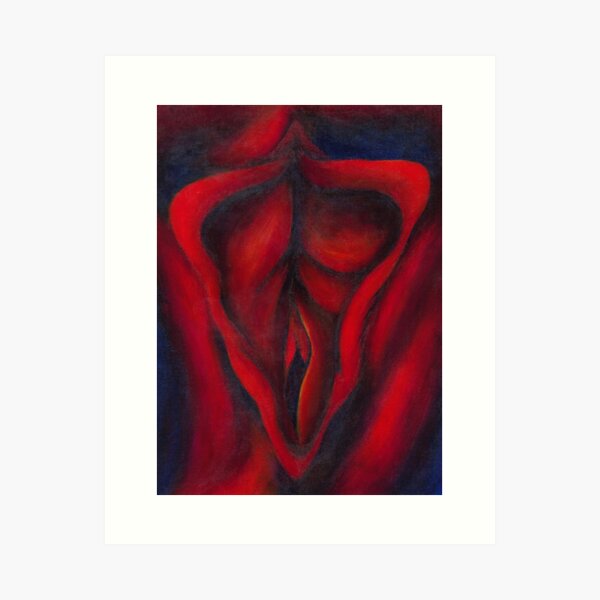This abstract painting features a vivid red, velvety triangular form that resembles an opening or possibly a flower, set against a striking combination of black and blue hues. The image presents a cave-like structure with curving lines, flaps, and asymmetrical shapes, creating a sense of depth and complexity. The lower part of the form has a darker tone with black accents, while the upper section incorporates hints of blue, enhancing the mysterious atmosphere. The quality of the photograph capturing the painting is not high, adding to its abstract and enigmatic nature. There is no signature or text to provide context, leaving the viewer to interpret the artist's intent through the rich, dark colors and dramatic contrasts in the composition.